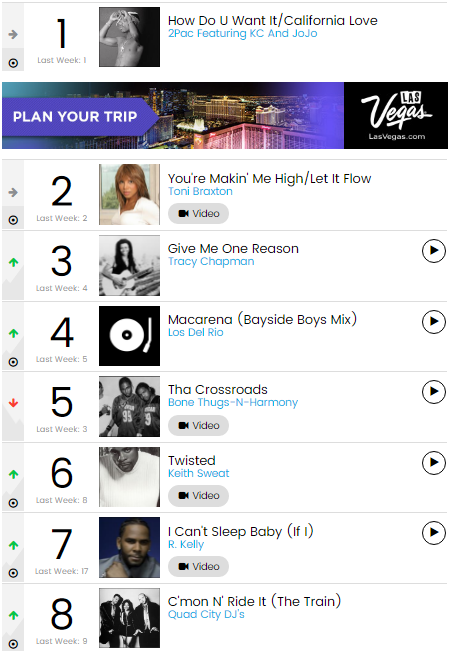This is a vertically-oriented smartphone screenshot displaying a music chart interface. A thin gray line borders the top and left sides of the image. Across the top, there are various small gray rectangles, each featuring icons such as arrows and a bullseye, including a green arrow pointing upwards, a red arrow pointing downwards, and a black bullseye.

On the left side of the image, the chart numbers are listed, showing both the current and previous week's rankings for each song. 

1. **"How Do You Want It / California Love" - 2Pac featuring K-Ci and JoJo**  
   Current position: #1 (Last week: #1)  
   The album cover is displayed next to the title. Below this entry, there's an ad recommending a trip to Las Vegas.

2. **"You're Makin' Me High / Let It Flow" - Toni Braxton**  
   Current position: #2 (Last week: #2)  
   The single's artwork is visible, along with a linked video.

3. **"Give Me One Reason" - Tracy Chapman**  
   Current position: #3 (Last week: #4)  
   Includes the song's cover art and a play button on the right side.

4. **"Macarena (Bayside Boys Mix)" - Los Del Rio**  
   Current position: #4 (Last week: #5)  
   Accompanied by the song's image and a play button.

5. **"Tha Crossroads" - Bone Thugs-N-Harmony**  
   Current position: #5 (Last week: #3)  
   Displays the cover image and a play button.

6. **"Twisted" - Keith Sweat**  
   Current position: #6 (Last week: #8)  
   Features the song's artwork, a video, and a play button.

7. **"I Can't Sleep Baby (If I)" - R. Kelly**  
   Current position: #7 (Last week: #17)  
   Comes with the cover image, a video, and a play button.

8. **"C'mon N' Ride It (The Train)" - Quad City DJ's**  
   Current position: #8 (Last week: #9)  
   Shows the track's artwork and a play button.

Overall, the interface is interactive and provides multiple links for playing videos and songs directly from the chart.